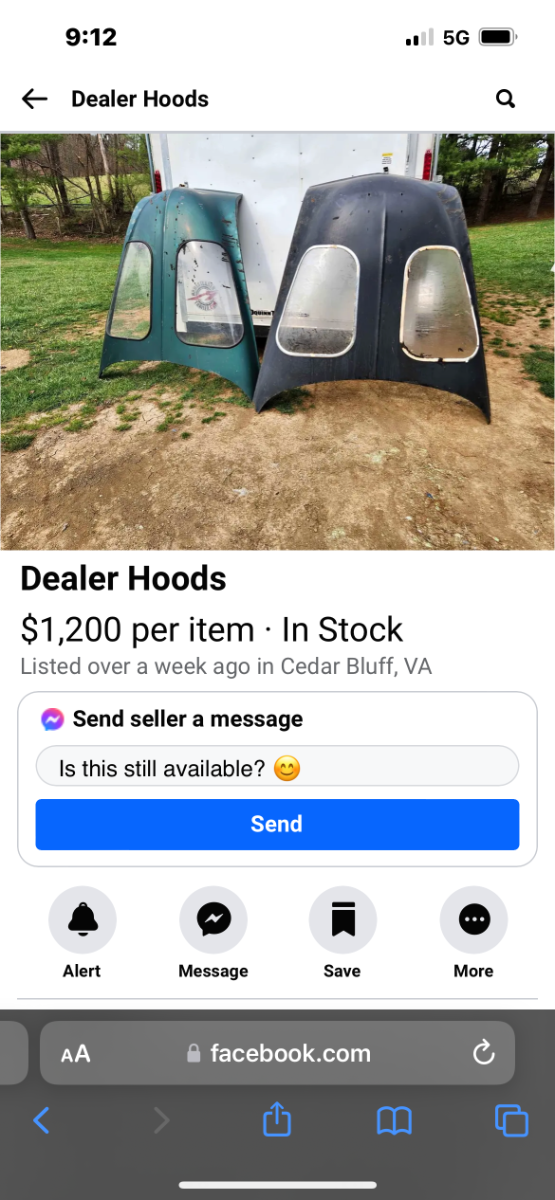This cell phone image captures a detailed screenshot of an online marketplace listing for vehicle hoods. The phone displays 5G connectivity with nearly a full battery charge at 9:12 AM. At the top of the screen, an arrow labeled "Dealer Hoods" points to the left, and a magnifying glass icon appears on the right for search functionality.

The listing features a clear photograph showing a grassy area with patches of dirt and a trailer holding two vehicle hoods in the foreground. One hood is a greenish color, while the other is black with see-through windows. The listing's details include a price of $1,200 per item, indicating they are in stock and were listed over a week ago in Cedar Bluff, Virginia.

Beneath the product information is a section for buyers to send a message to the seller, including a prompt to inquire, "Is this still available?" with a clickable button featuring a smiley face. At the bottom of the screen are circular icons for alert, message, save, and more options, followed by the Facebook logo link.